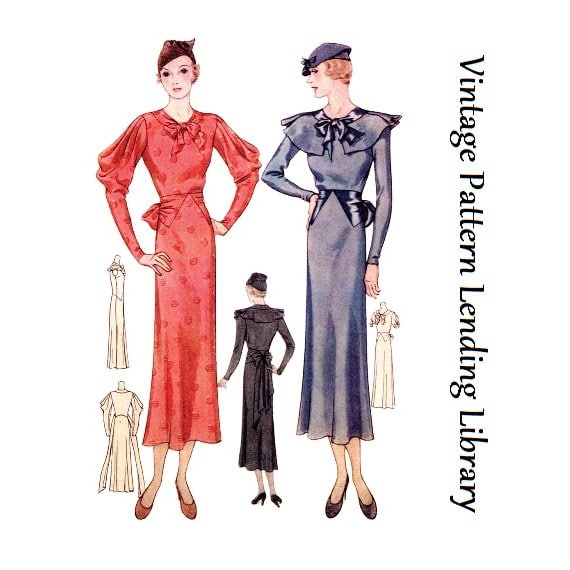The image depicts an early 20th-century fashion magazine sketch, likely dating between 1910 and 1920. Dominating the center are two elegantly dressed women in ankle-length gowns. The woman on the left is adorned in a light red or pink dress with long sleeves, featuring a ribbon or bow at her collar, and she sports matching red shoes. Her hands rest confidently on her hips beneath a small hat. To the right, another woman is captured in a blue dress with a large bow on both her collar and waist, paired with matching shoes. She is glancing towards the woman on her left, with one hand on her hip and the other relaxed by her side. Positioned in the background is a third woman in black attire, her back turned to the viewer, highlighted by a bow at her waist, and also wearing black shoes. Surrounding them are schematic sketches of dresses on a cream background, adding to the vintage aesthetic. The right side of the picture bears the text "Vintage Pattern Lending Library" in elegant calligraphy, enhancing the nostalgic feel of the artwork.